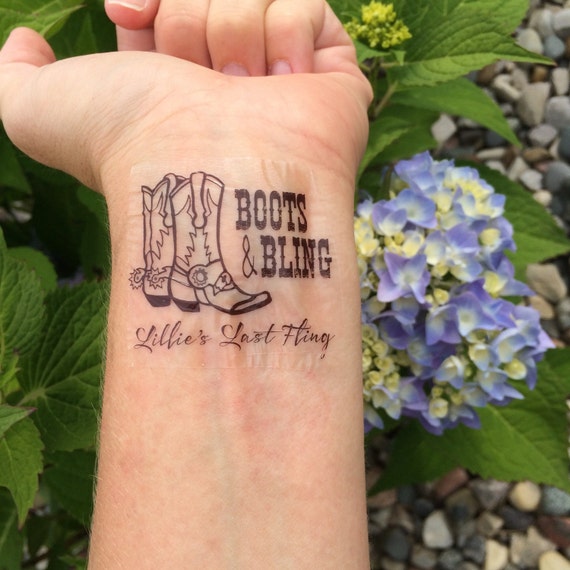The square image centrally features a Caucasian person's left wrist, holding their hand in a bent position, thumb pointing left and fingers curled downward. On the wrist is a temporary, transparent tattoo sticker with a visibly clear outline. The tattoo displays two pairs of cowboy boots and the text "Boots and Bling" in an old west font, accompanied by the cursive phrase, "Lily’s Last Fling." The tattoo, primarily in black ink, contrasts the vibrant outdoor backdrop, which includes purple and cream flowers and lush green leaves, set against pebbles on the ground. The hand's positioning and the intricate details of the tattoo, juxtaposed with the natural elements, create a visually arresting scene imbued with a sense of whimsy and temporary charm.